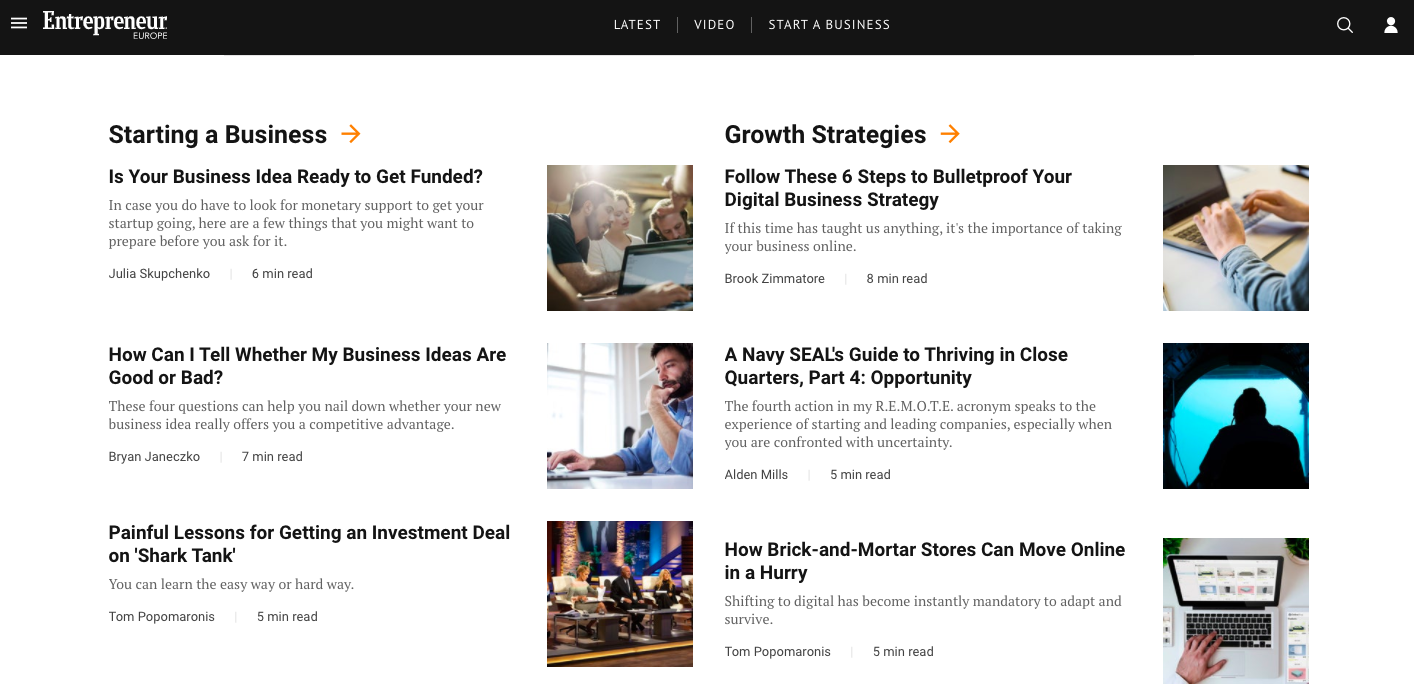**Detailed Caption:**

This image features a section of the Entrepreneur website, prominently branded in white text located in the top-left corner against a solid black background. The top section of the image is predominantly black. Positioned in the center under the top section are three small written categories. In the top-right corner, there are two icons—a search icon and a profile icon.

The layout of the image is divided vertically into two main sections: "Starting a Business" on the left and "Growth Strategies" on the right. Each section features three articles, all accompanied by square images to the right of their titles.

On the left side, under the heading "Starting a Business," marked with an orange arrow pointing to the right, we have the following articles:
1. "Is Your Business Idea Ready to Get Funded?" 
2. "How Can I Tell Whether My Business Ideas are Good or Bad?" 
3. "Painful Lessons for Getting an Investment Deal on Shark Tank."

On the right side, under the heading "Growth Strategies," similarly marked with an orange arrow pointing to the right, are:
1. "Follow These Six Steps to Bulletproof Your Digital Business Strategy."
2. "A Navy SEAL's Quick Guide to Thriving in Close Quarters: Part Four - Opportunity."
3. "How Brick and Mortar Stores Can Move Online in a Hurry."

The entire section is set against a white background, providing a clean and organized layout for easy reading.